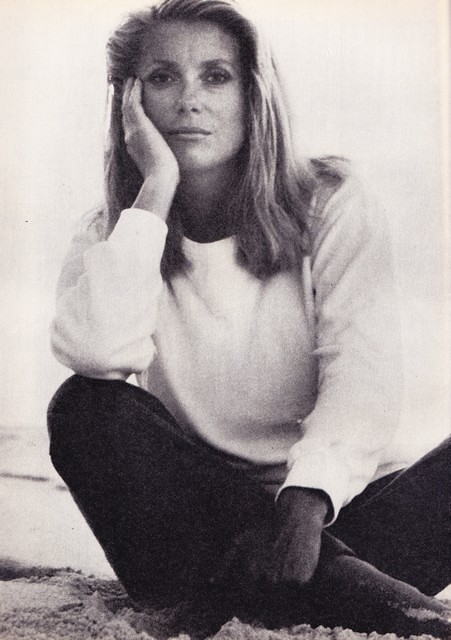This black and white photograph features a woman sitting contemplatively on a sandy surface, looking directly at the camera with a serene expression. Her straight hair, which appears darker at the roots and lighter towards the ends, falls about four inches below her shoulders and is slightly pulled back. She wears a light-colored long-sleeved sweater paired with dark pants. Her right hand supports her cheek and chin while her left hand rests on her ankle. The background is a pure, blurred white, giving the impression of being outdoors though it's ambiguous. The overall composition provides a serene, almost timeless quality to the image.